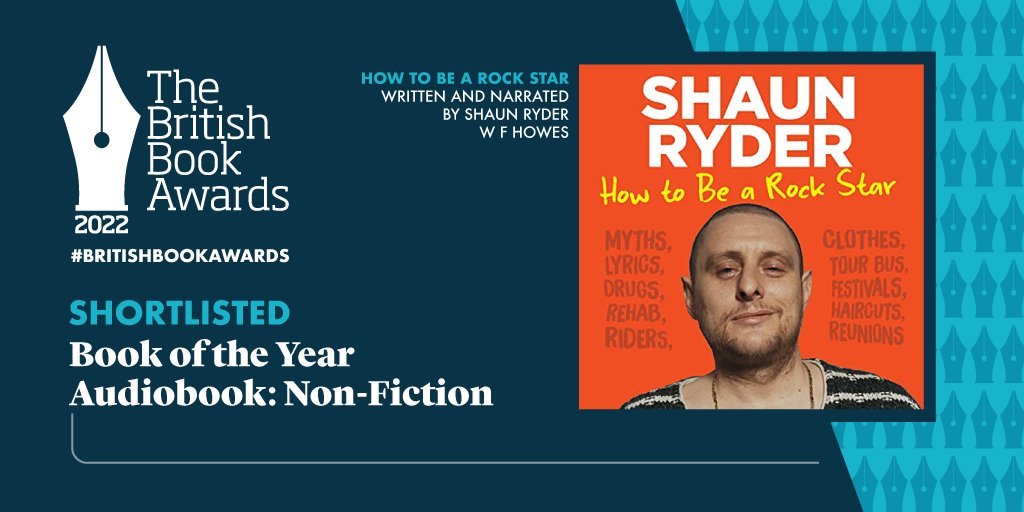The image is an advertisement for the audiobook "How to Be a Rock Star" by Shaun Ryder, which has been shortlisted for the British Book Awards in 2022. The background is divided with a dark blue on the left and a light blue on the right, overlaid with the audiobook's cover image. Shaun Ryder's name appears in white capital letters at the top of the cover, along with the title "How to Be a Rock Star" handwritten in yellow. On the left-hand side, the British Book Awards logo, depicting an old-style ink pen tip, is prominently featured in white. Below the logo, the text reads "2022" and "#BritishBookAwards". Additionally, phrases like "shortlisted," "Book of the Year," and "Audiobook: Non-fiction" appear in blue and white. The cover also includes a photo of Shaun Ryder’s head and shoulders against an orange backdrop, accompanied by keywords like "myths, lyrics, drugs, rehab, writers, clothes, your bus, festivals, haircuts, reunions" in dark orange text. At the bottom, it declares the audiobook is "written and narrated by Shaun Ryder" and is produced by WFHOWS.